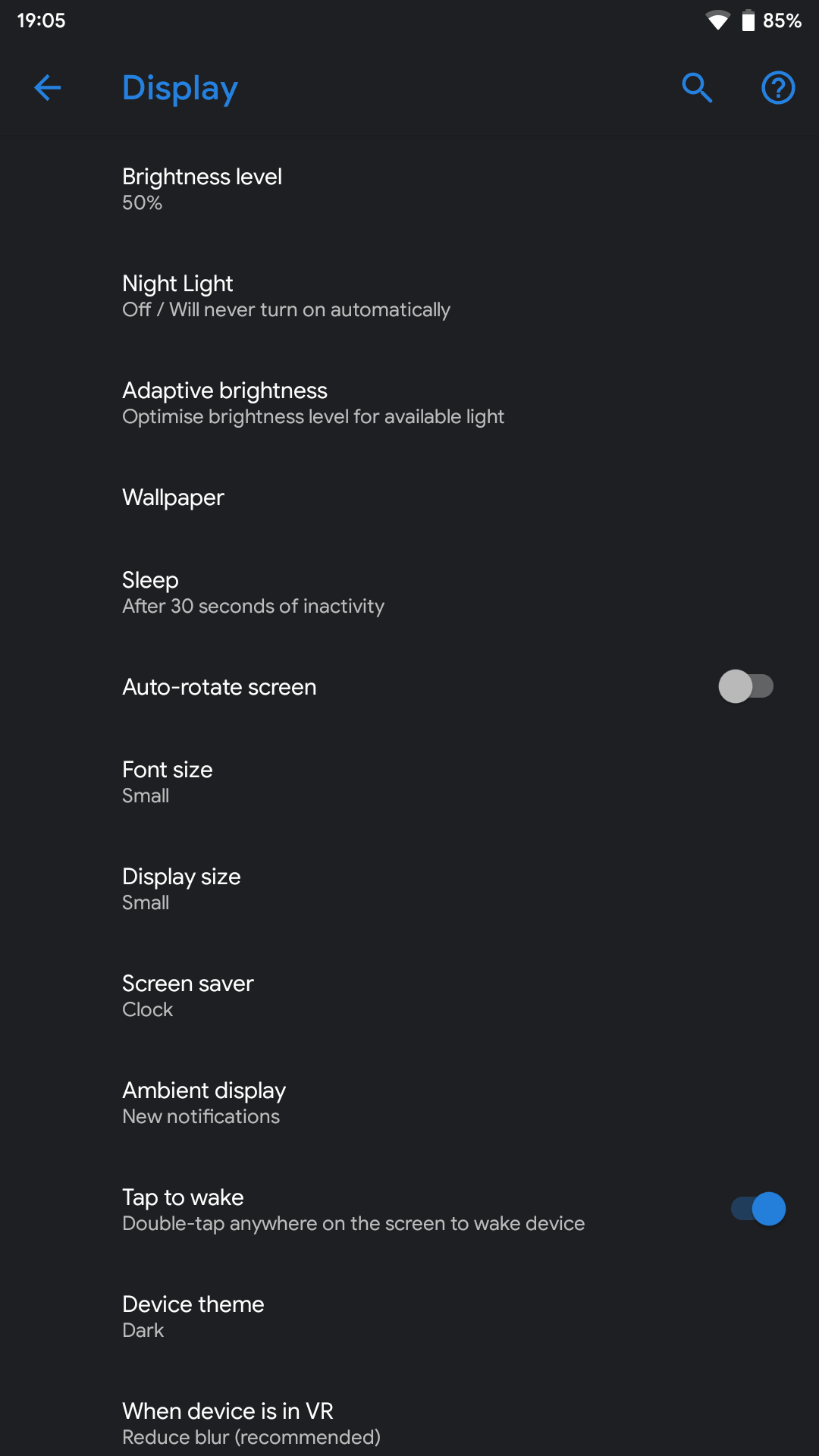Screenshot of a device display settings menu against a black background, featuring a blend of white and blue text. The upper left corner shows the time as "19:05" in white text. On the upper right, icons for Wi-Fi and battery status (at 85%) are visible. Directly below, blue icons for a left arrow and a magnifying glass are displayed. In smaller white text, it indicates the "Brightness level: 50%," followed by "Night Light: Off" with a note that it "Will never turn on automatically." The setting "Adaptive brightness," highlighted in bold white text, is described as optimizing "brightness levels for available light." The menu continues with "Sleep after 30 seconds of inactivity" and "Auto-rotate screen," the latter of which has a toggle switch shown in the off position. Further down, options for "Font size: Small," "Display size: Small," "Screen saver: Clock," and "Ambient display" are listed. The "Tap to wake" function is explained as "Double tap anywhere on the screen to wake device," with the accompanying blue toggle switch in the on position.